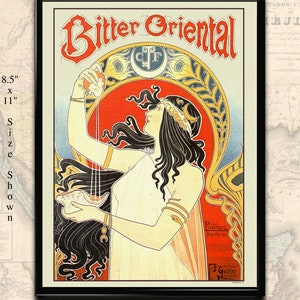The color photograph displays an intricately detailed painting over a wall, resembling a framed piece with an ivory background. Dominating the top section of the painting is the title "Bitter Oriental" in striking red letters. The central figure in the artwork is a woman depicted with long, flowing black hair, adorned in a white toga-like dress that drapes off her shoulders. She is accessorized with several bracelets, including a distinctive snake-shaped arm band encircling her upper arm and a golden wrap elegantly placed around her head. 

The woman is posed gracefully, with one arm raised above her head while the other is held out in front of her chest, clutching a shell. A trio of white strings connects her extended arms, descending inward. Above her head, an ornate golden arch adds to the mystique of the scene. The background features a faint outline of a map, enhancing the depth and context of the image. Along the left side of the photograph, there are black letters indicating the dimensions, “eight and a half by eleven size shown,” further grounding the piece in a real-world context. The artwork's vibrant palette of red, yellow, and black contrasts beautifully, making the imagery and typography stand out.